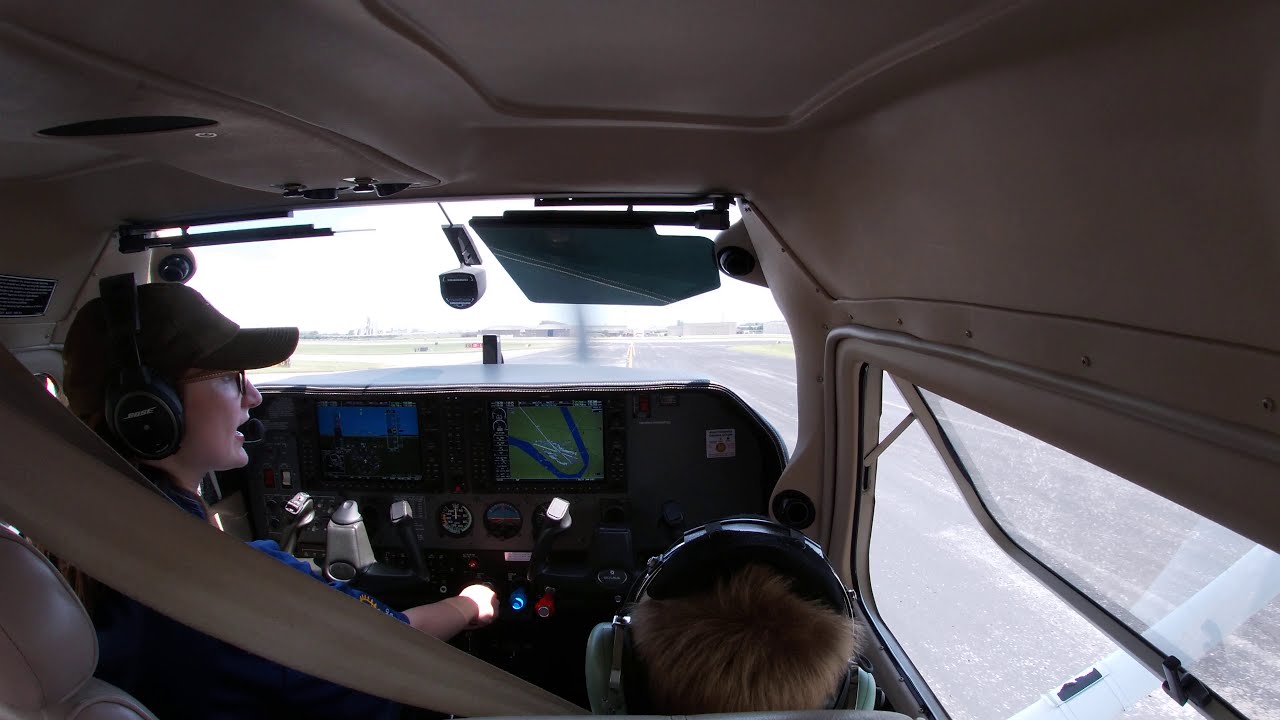In this detailed image, we find ourselves inside the modern cockpit of a small propeller plane during the day. Dominating the left side of the frame is a Caucasian woman, identifiable by her black baseball cap, glasses, and black Bose headphones. She is seated at the left yoke, her hand engaged with the digital controls on the console before her, which includes a green display, likely a GPS or map tracker. Seated next to her at the right yoke is a young boy, discernible by his smaller stature and brown hair, wearing gray headphones for ear protection. Both individuals are securely strapped in with seatbelts. A window to their right provides a clear view of the plane's metal wing extending out, with the tarmac and runway visible beyond. The cockpit itself is a mix of tan leather and digital displays, suggesting a blend of traditional and contemporary aviation technology. The scene captures a focused moment of piloting, enhanced by the blurred motion of a propeller blade visible through the windshield.